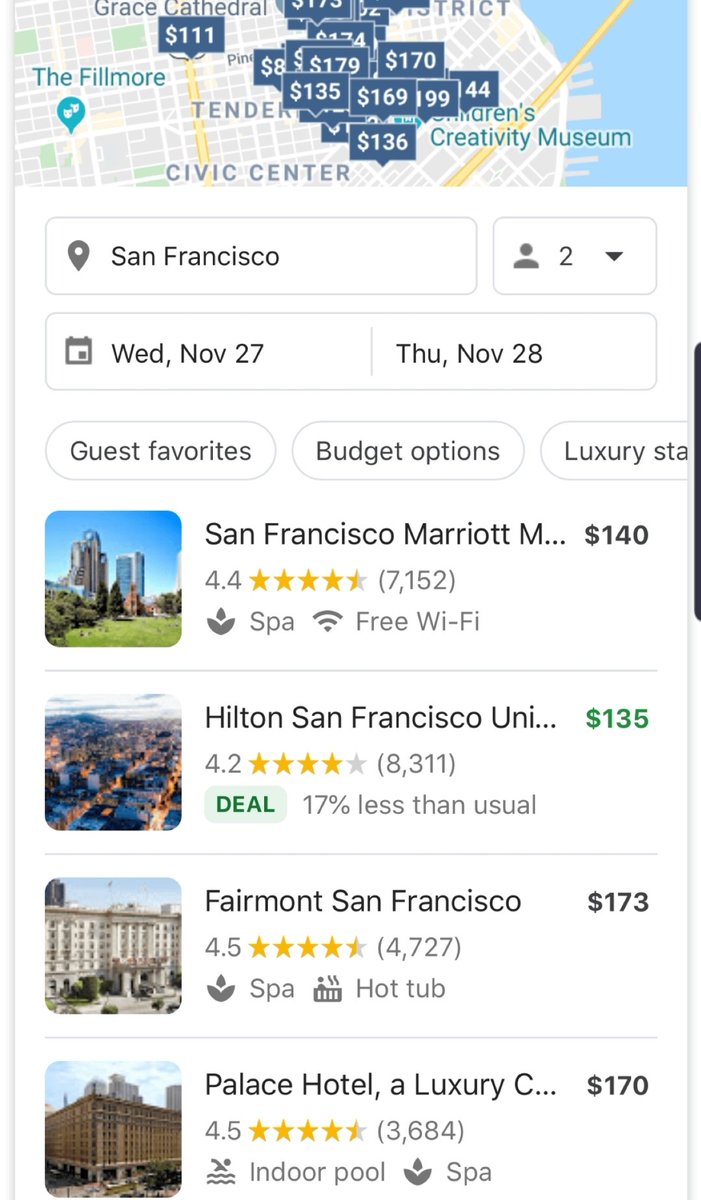This image depicts a screenshot from a smartphone app, which appears to be designed for booking hotel reservations. At the top of the screen, there's a band featuring a partial map of San Francisco, cluttered with overlapping blue boxes displaying various hotel prices, such as $136, $169, and $179. Due to the overlap, individual hotels and corresponding prices are indistinguishable unless the map is zoomed in on.

Beneath the map, there are input boxes where users have specified their destination as San Francisco, along with their arrival and departure dates. To the right of the city box, there's another box indicating the number of people in the party, marked as two in this instance.

The main content area lists four hotel options, all located in San Francisco. The first hotel listed is the San Francisco Marriott, priced at $140 per night. The second is the Hilton San Francisco, priced at $135 per night. The third hotel shown is the Fairmont San Francisco, with a nightly rate of $173. The fourth entry is the Palace Hotel, listed at $170 per night. Additionally, each hotel listing is accompanied by various icons denoting amenities such as spas, hot tubs, indoor pools, and free Wi-Fi.

The page is not displayed in its entirety, as indicated by the visible scroll bar on the right side, suggesting more content is available further down.